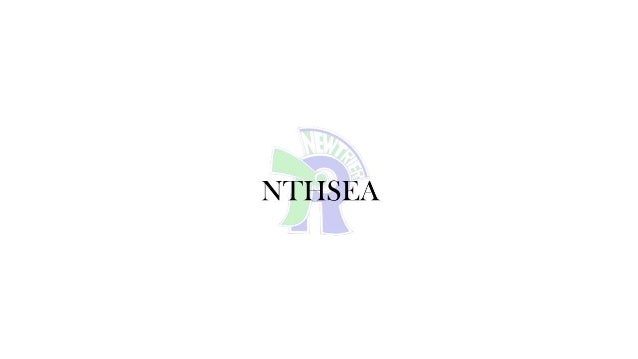The image is a minimalist depiction featuring what appears to be a company logo, centrally positioned against a solid white background. Dominating the foreground is bold, black text spelling out "N-T-H-S-E-A" in all capital letters. Behind this text, a somewhat abstract and faded logo blends into the background, making it difficult to discern specific details. The logo incorporates a green shape resembling the number 7, overlapping with a purple element that takes on the form of an R. Within the circular part of the R, positioned towards the top right, there is white text that reads "NEW TRIER" in all caps, set against the same green color as the 7 and featuring a thin purple border. Colors present in the image include white, black, green, and purple. The overall composition suggests a design that could be used for a business card or corporate website.